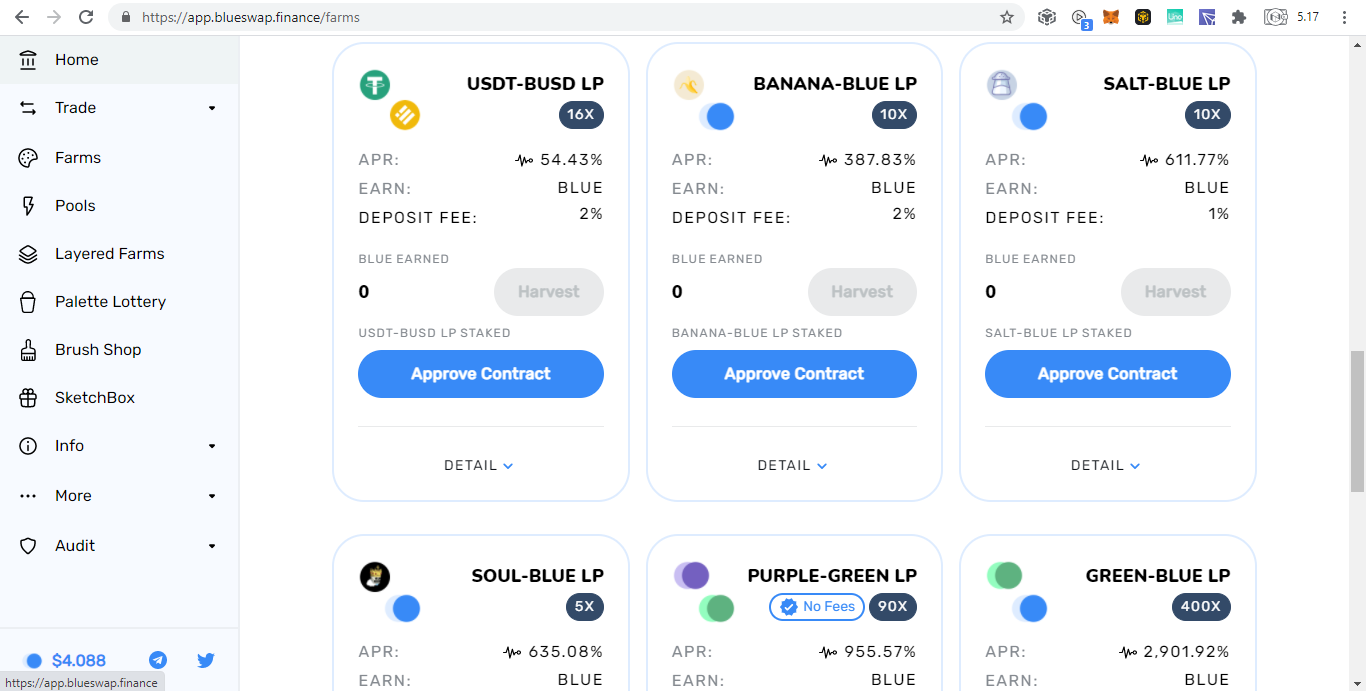Screenshot of a finance-related website, potentially titled "Blueswap Finance," as indicated by the partial URL visible at the top of the image (app.blueswap.finance). The interface displays six informational cards, with the top three fully visible and the bottom three partially cut off.

1. **First Card:**
   - **Title:** USDT BUSD LP
   - **Amplification Factor:** 16x
   - **APR:** 54.43%
   - **Earnings:** Earn Blue
   - **Deposit Fee:** 2%
   - **Action Buttons:**
     - **Green Button:** Harvest
     - **Blue Button:** Approve Contract
   - **Details:** At the very bottom, a "Detail" label with a blue downward-pointing arrow.

Each card shares the same layout and design, with corresponding buttons and details presented in a structured format. The overall design suggests functionalities related to finance and investment, such as liquidity provision, earnings, and contract approvals.